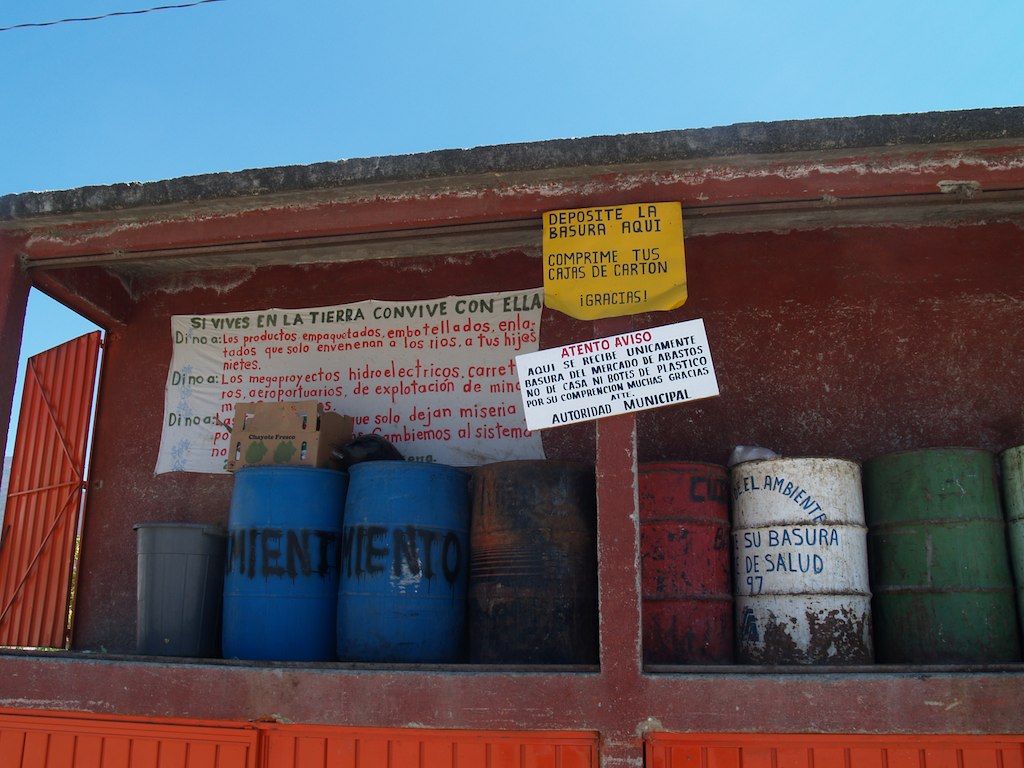In this image, we see the interior of a worn, dark red structure located at the top of a building. The room has an open door on the left side, revealing a glimpse of the sky. Within this rustic and dirty space, barrels are stacked in a row. Starting from the left, there's a gray plastic trash can, followed by two blue barrels with black, spray-painted Spanish text. Next, there's a rusted barrel with a dark, orange-gray hue. To the right of this rusty barrel, there are more containers: a red barrel, a white barrel with blue Spanish lettering, and finally, two dark green barrels. 

On the wall to the left side above the barrels and trash can, hang three signs, all written in Spanish. The top sign is yellow and reads, "Deposite la basura aquí. Comprimidas cajas de cartón. Gracias." Below this, another sign features black and red spray-painted text, largely obscured by the barrels. The last one is an attention sign. The overall ambiance is one of neglect and decay, with the building’s metallic framework adding to the grimy and industrial appearance.